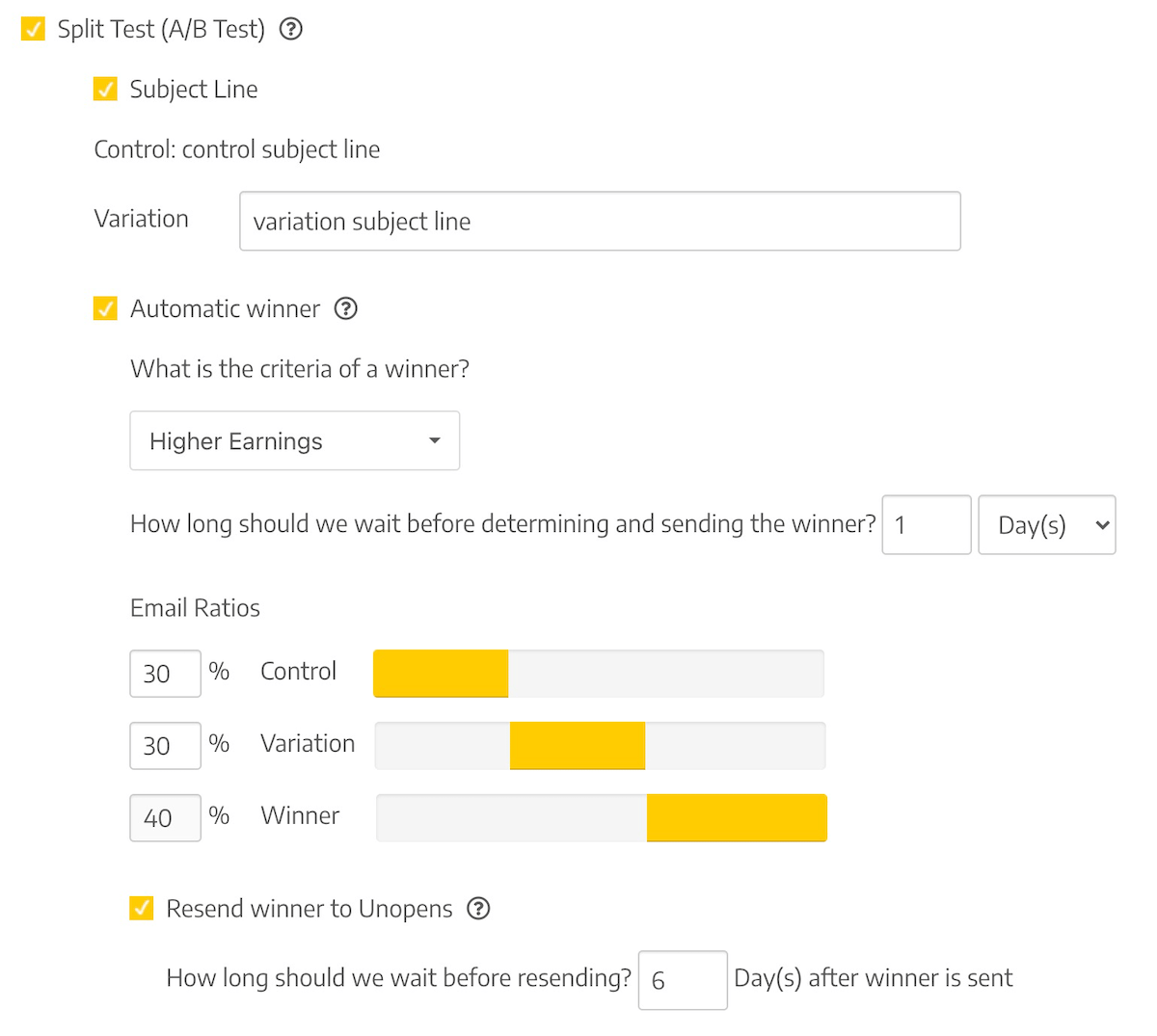This screenshot displays a website interface focused on setting up an email split test campaign. In the top left corner, it reads "Split Test" with an associated label "A/B Test." Below this, there's a section titled "Subject Line," divided into "Control Subject Line" and "Variation Subject Line" fields. An additional feature, "Automatic Winner," appears with specified win criteria based on "Higher Earnings."

Further down, a question asks, "How long should we wait before determining and sending the winner?" with the selected option being "1 day." The "Email Ratio" section indicates a distribution of 30% for the Control group, 30% for the Variation group, and 40% for the Winner.

A secondary instruction reads, “Resend to Unopens," followed by "How long should we wait before resending?" with a set duration of "6 days after the winner is sent." This suggests the campaign includes a follow-up strategy for unopened emails, implementing a six-day waiting period before resending. Overall, the setup appears designed for optimizing email marketing effectiveness through a structured A/B testing approach.